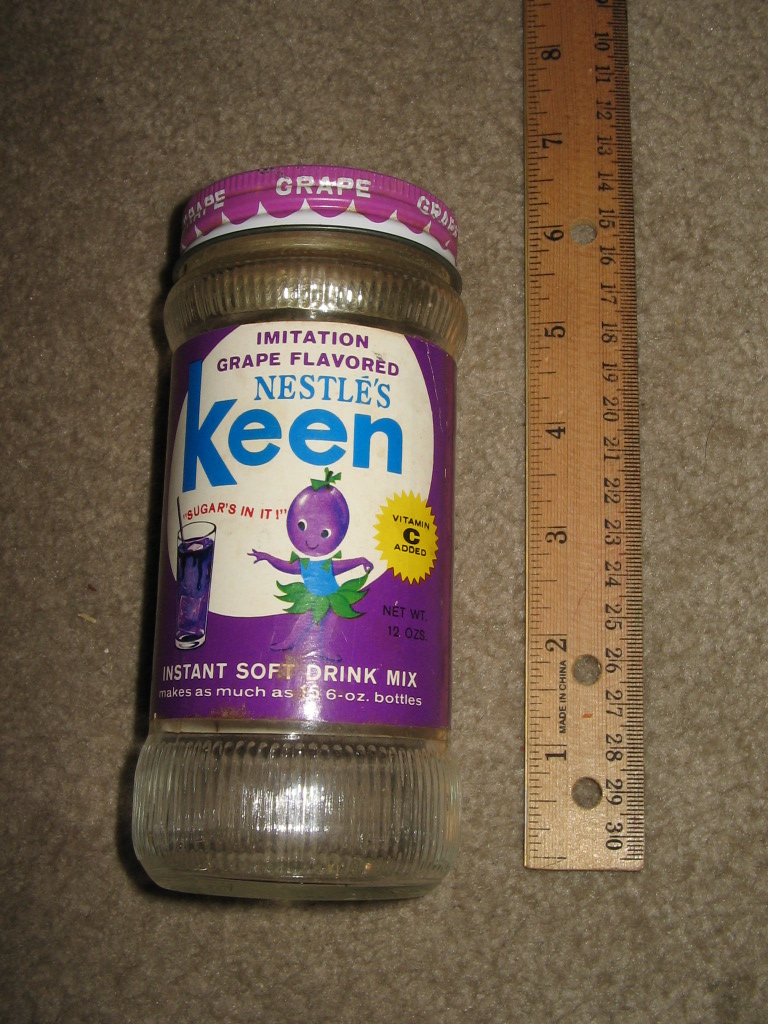The photograph features a vintage, empty glass jar of Nestle's Keen Instant Soft Drink Mix, lying on its side atop beige carpeting. The jar, which is around 6 inches tall and 3 inches wide at its broadest part, is positioned next to a brown wooden ruler for scale. The textured glass jar has a smooth section in the middle where its vibrant purple and white label resides. The label prominently displays "Imitation Grape Flavored" and "Instant Soft Drink Mix," noting it can make as much as sixteen 6-ounce bottles of drink. Additionally, it mentions that the product contains sugar and has added Vitamin C. The jar is topped with a purple, metal screw-on lid that says "Grape" in white. The label also showcases a charming cartoon character, a grape dressed in a green skirt and blue blouse, pointing at a cup of grape drink.